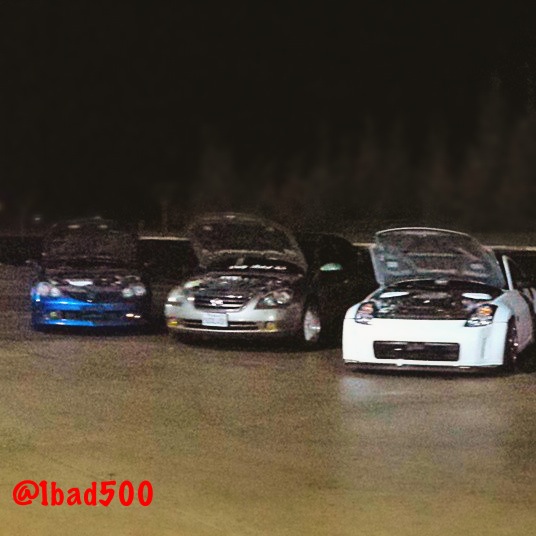This nighttime photograph captures three sports cars on display in an outdoor parking lot, their hoods open and facing directly at the camera. The scene is dimly lit, with faint outlines of trees in the background against the dark sky. The concrete ground exhibits darker tire marks in circular patterns, hinting at possible donuts. In the lower left-hand corner, red text reads "AT 1 BAD 500." The lineup of cars includes, from left to right, a metallic blue car, a metallic silver car with silver rims and a front license plate, and a white car featuring a black grille and chrome wheels.